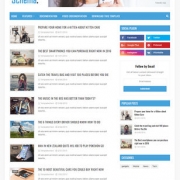The image is quite blurry and extremely small. In the upper left corner, there is some blue text about two inches long, but it is unreadable. Below this, there is a long blue rectangle approximately six inches in length with small, blurry, and illegible white text inside. 

The main section of the image contains seven squares, each about two inches in size, depicting various scenes. In the second square, there appears to be someone leaning against a yellow car. The third square shows a girl with brown hair. Moving downward, one of the squares features green grass with a backdrop of blue sky and white clouds. Below that, another square seems to display a white tent. The final square in this section seems to show an iPad lying on a table.

On the right side of the image, there is a column of rectangles, which seem to represent different social media platforms. The colors used suggest purple for Instagram, light blue for Twitter, navy blue for Facebook, and red for Pinterest.